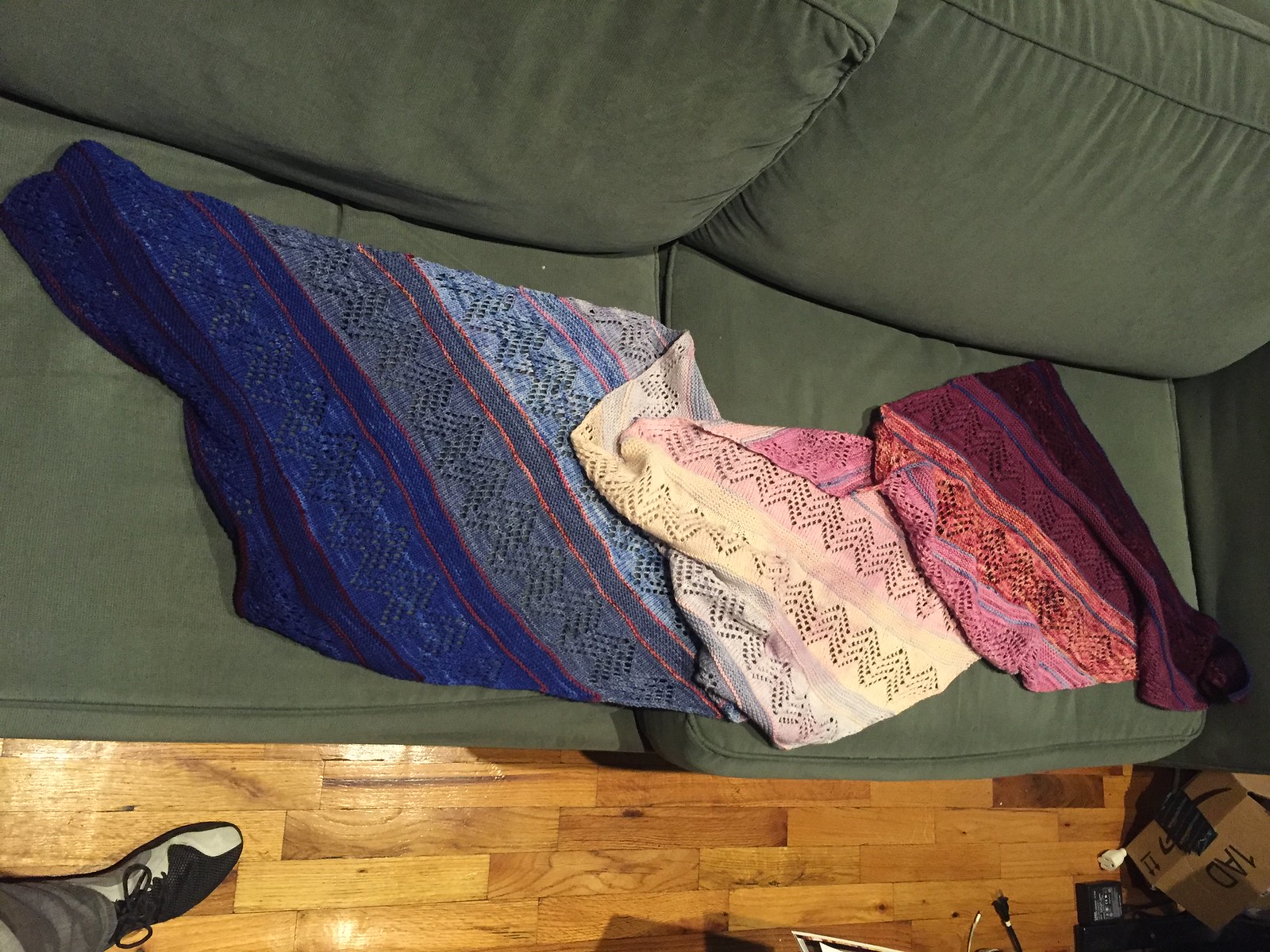The image is a color photograph taken from a nearly first-person, bird's-eye view. At the bottom of the frame, the right foot of the person taking the photo is visible, clad in a shoe that is black with a light grey stripe and black laces. The person is standing on a wooden floor comprised of horizontal parquet panels, varying in tone from dark brown to light mahogany. 

In front of the person is a green material couch, with its seat and back cushions in view. On the seat cushions, there are three separate pieces of cloth, which appear to be head scarves. These pieces of cloth are crumpled and not fully spread out, showing different colors and designs. The cloth on the right features a mix of light purple, orange, reddish, and dark brown hues. The middle cloth has a yellow and light pinkish color, adorned with a zigzag pattern. The piece on the left displays a combination of dark blue, grey, blue, and lighter grey dotted patterns, intersected by red lines.

In addition to these elements, a brown box, possibly from Amazon, is situated to the right near the couch. The overall setting includes a green couch on a richly toned wooden floor, with vibrant, patterned cloth pieces creating a visually stimulating scene.